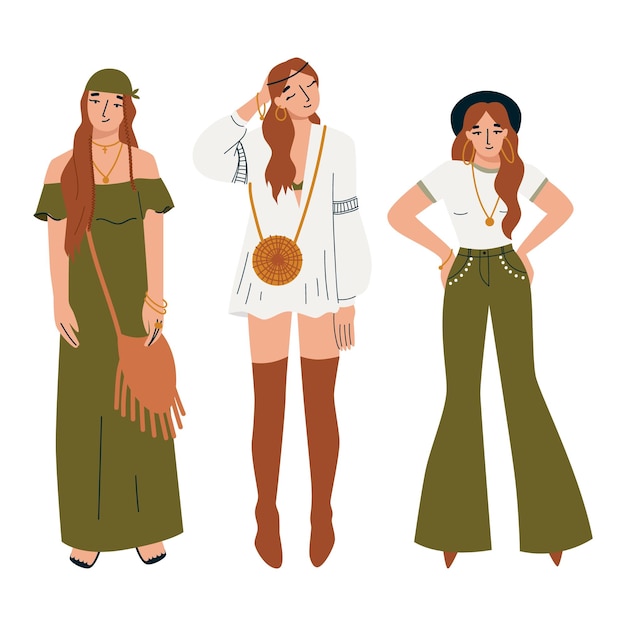In the illustration, three women are depicted in detailed and colorful attire. The woman on the left is adorned in a shoulderless green dress that flows down to her feet, with bare feet visible. She accessorizes with a green bandana tied around her head, long dark brown hair cascading down in braids, two bracelets, and layered necklaces. A light brown fringed purse hangs across her body from her right shoulder. The woman in the middle stands out with her white, long-sleeved, V-neck shirt accented with blue details, and reddish colored high boots. She has a brown crossbody bag slung from her left shoulder to her right side, a black band across her forehead, and a bracelet on her right wrist. Her right hand is posed on the back of her head, and her eyes are closed. The woman on the right is slightly shorter, dressed in a white top paired with long green pants and pointy brown shoes. Her look is completed with a black hat, big hoop golden earrings, a golden necklace, and a bracelet on her right wrist. Each woman showcases distinctive yet complementary fashion styles, with a mix of detailed accessories that highlight their individual yet cohesive appearances.